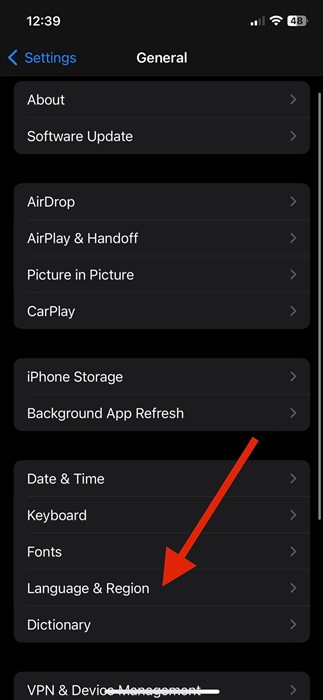This is a detailed screenshot of a smartphone's Settings page with a dark theme. The background is entirely black, and each menu option is set against light or dark gray backgrounds.

At the top of the screen:
- The current time is 12:39 PM.
- There are two bars indicating internet connectivity.
- The battery is at 48%.

Below this, the header section displays:
- "Settings" in blue, accompanied by a blue caret pointing to the left.
- The title "General" is centered below the header.

The menu is divided into four main sections:

**First Section:**
1. "About" with a caret pointing to the right.
2. "Software Update" with a caret pointing to the right.

**Second Section:**
1. "AirDrop" with a caret pointing to the right.
2. "AirPlay & Handoff" with a caret pointing to the right.
3. "Picture in Picture" with a caret pointing to the right.
4. "CarPlay" with a caret pointing to the right.

**Third Section:**
1. "iPhone Storage" with a caret pointing to the right.
2. "Background App Refresh" with a caret pointing to the right.

**Fourth Section:**
1. "Date & Time" with a caret pointing to the right.
2. "Keyboard" with a caret pointing to the right.
3. "Fonts" with a caret pointing to the right.
4. "Language & Region" with a caret pointing to the right, highlighted by a red arrow indicating that this option has been selected or is of particular importance.
5. "Dictionary" with a caret pointing to the right.

At the bottom of the visible screen, there’s the start of another section that includes "VPN & Device Management" with a caret pointing to the right, although the rest of this section isn't fully visible in the screenshot.